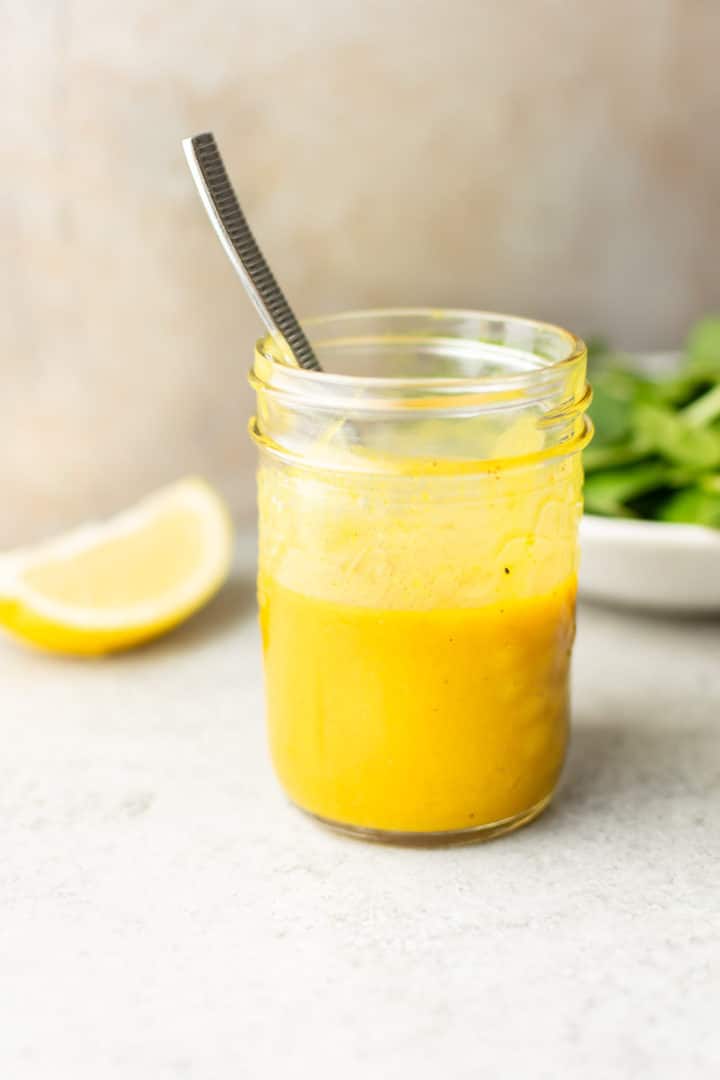The photo is a vertically aligned rectangular image featuring a glass jar about half full of a dark yellow liquid, presumably a sauce. The jar, which is a clear glass cylinder with ridges around the rim, is accompanied by a silver utensil, likely a spoon, inside it. Positioned to the left middle side, partially behind the jar, is a slightly blurry lemon wedge. To the right in the background is a white dish filled with green leaves or possibly broccoli, adding to the photo's depth. The marbled surface on which the jar rests is predominantly white with streaks of gray, enhancing the overall composition. Completing the scene, the blurred backdrop appears to be a blend of brown and white stone, creating a warm, cohesive ambiance.